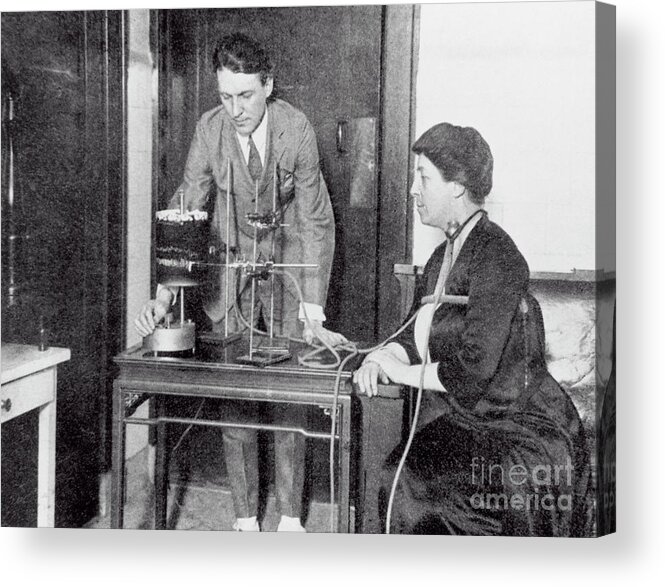This black and white canvas-printed photo captures a historical scene featuring a man and a woman, likely from the Industrial Age, amidst what appears to be scientific or medical equipment. The man, dressed in a suit, is standing slightly off-center to the left, leaning over a wooden table with his left hand, while his right hand adjusts a complex instrument on the table. This instrument comprises cylindrical contraptions, interconnected rods, crossbars, and various tubes. These tubes extend and attach to the seated woman on his right. The woman, who has her hair pinned up and appears older, has some wires or tubes around her chest and her arm resting on the table. Behind the man, the setting includes a door, with another door and the corner of a white table visible on the far left of the image. The woman seems to be an integral part of the apparatus, indicating the possibility of a scientific experiment or medical procedure being depicted. The photograph includes a 3D border on the right side, enhancing the image's depth.